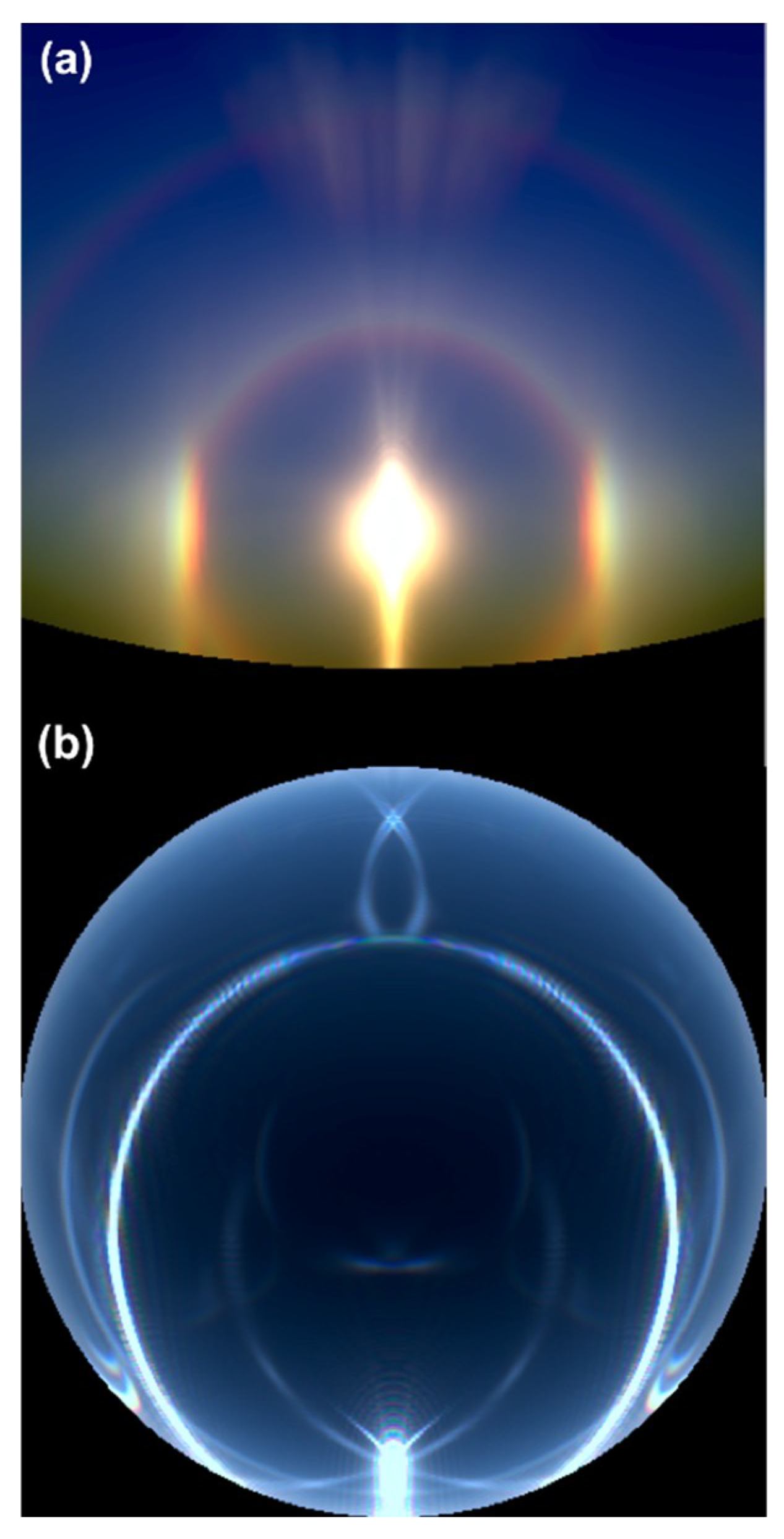This photo presents two vertically aligned images labeled A and B. The top half, labeled A, is dominated by a blue background with a striking bright yellow center that radiates a golden-orange aura, resembling a close-up view of an illuminated light bulb filament. Light beams extend upwards, creating a faint rainbow effect around this luminous core. The bottom half, labeled B, features a contrasting black background with a translucent blue orb at the center. This orb showcases intricate circular line patterns, illuminated by a radiant, whitish-blue light at its base. The predominant colors transition from the orangish hues in the upper section to the cooler blues in the lower section, tying the elements together in a visually compelling composition.